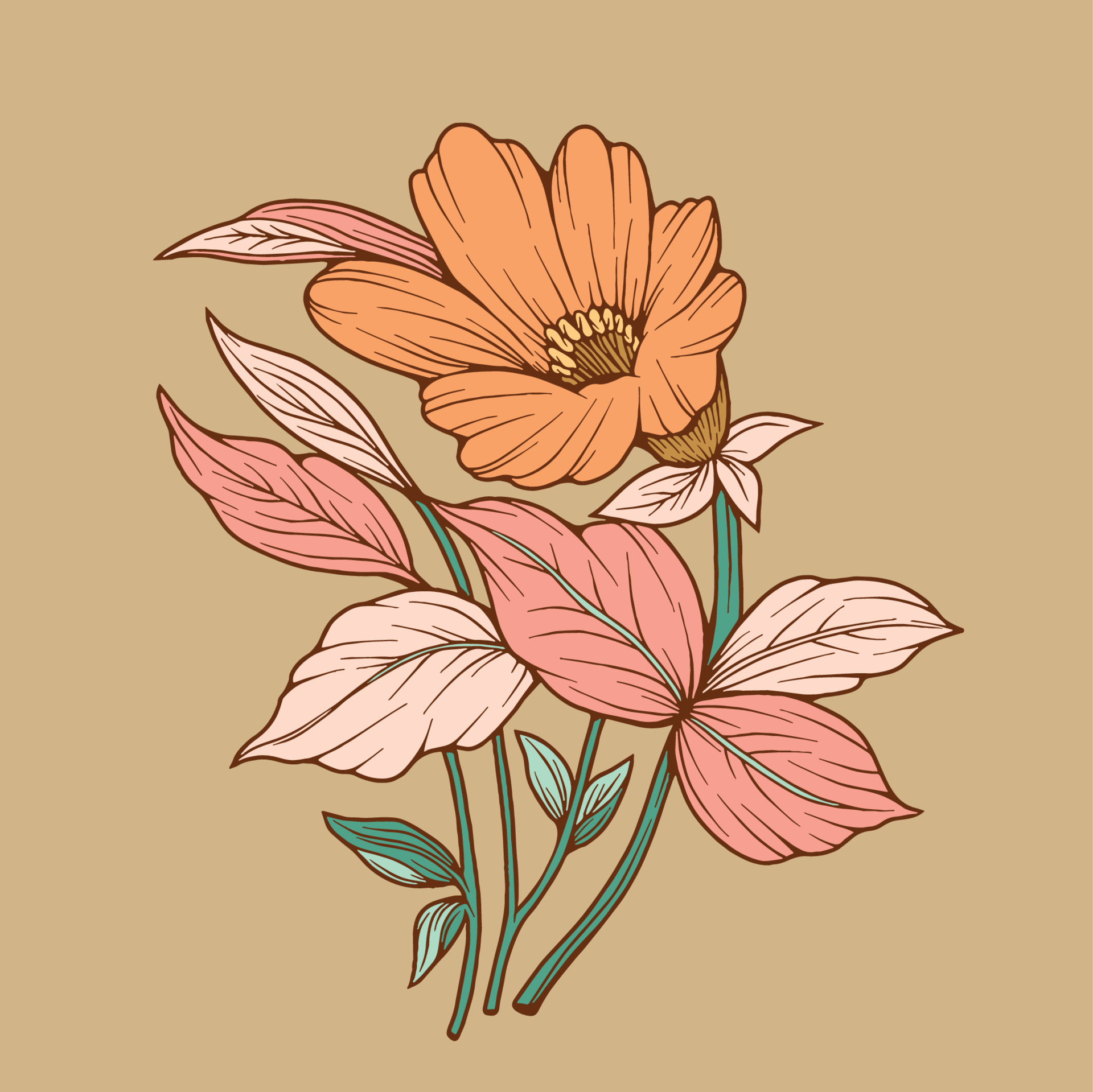The image is a square, about six inches in both height and width, with a light tan or light brown background. In the center, three green stems rise from the bottom of the image. The left stem features two small green leaves near the bottom and is partially obscured at the top, which might end with a large pink leaf. The central stem splits into two branches towards the left and right. The rightmost stem is the thickest, adorned with large, pink to almost light pink leaves. At its tip, an orange flower with yellow in the center, showcasing detailed petals and lines, stands out. The overall illustration appears to be a computer-generated graphical drawing of flowers.